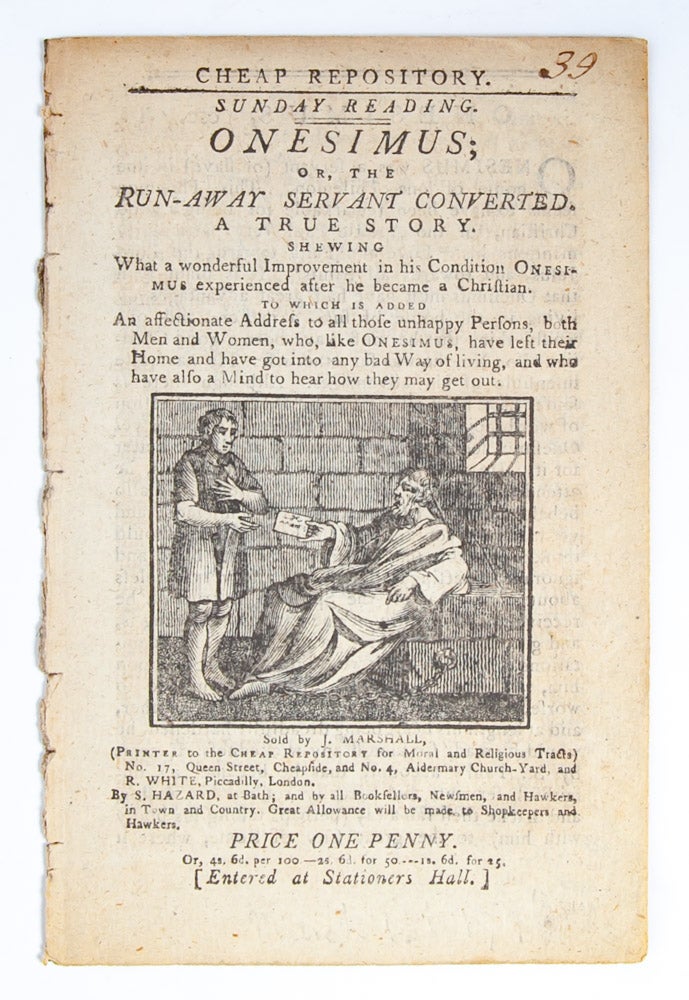The image is a photograph of an aged, torn-out page from an old book or possibly an old magazine, set against a white background. The left edge of the paper is jagged, indicating it was ripped from its original binding. At the top, the page prominently declares in dark colored font, "CHEAP REPOSITORY" with "SUNDAY READING" followed by "ONESIMUS OR THE RUNAWAY SERVANT CONVERTED" underneath, all capitalized. Below this header, it states "A True Story" and begins the narrative with two paragraphs of text.

Centrally positioned on the page is a grayscale illustration resembling an etching or engraving. This illustration depicts a nobleman in a light-colored robe, sitting and leaning against steps, handing a note to a barefoot servant who stands with one hand on his chest and the other reaching for the note. This visual is framed in a square and further illustrates the story. At the bottom of the page, it reads "PRICE ONE PENNY" followed by an additional paragraph of descriptive text.